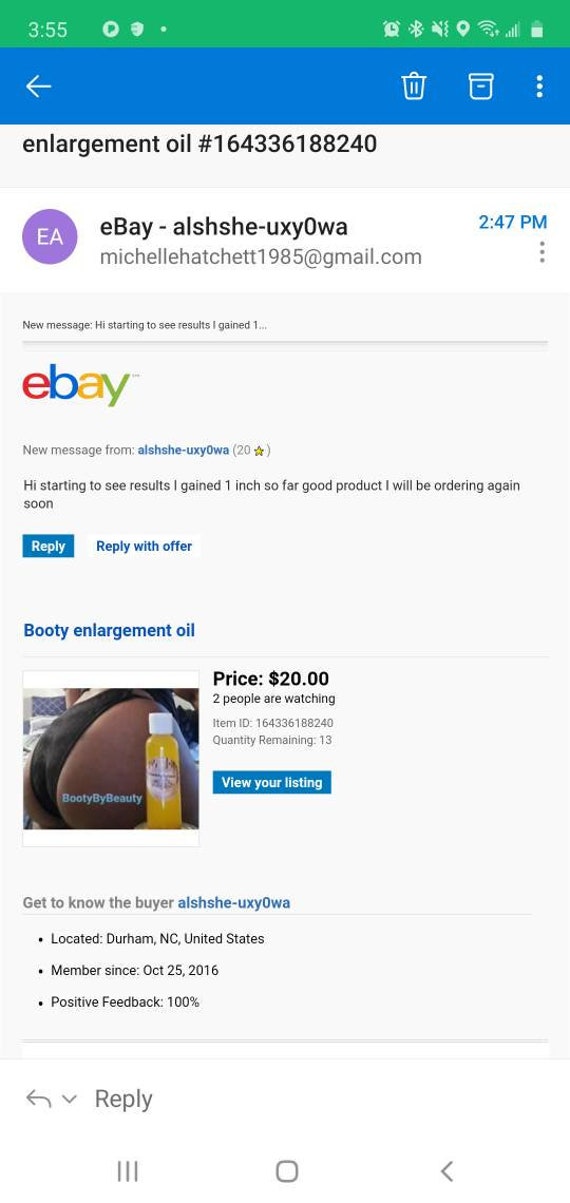**Detailed Caption:**

This is a smartphone screenshot depicting an eBay page. At the top, there is a green status bar featuring a timestamp "3:55," followed by various icons: a Pinterest logo, an unidentified shield logo, a clock icon, a Bluetooth icon, a sound icon (muted), a location icon, a Wi-Fi icon, and a battery icon. Below this status bar is a blue navigation section containing a left-facing arrow on the left margin, a trash can icon on the right, a container icon adjacent to it, and three vertical dots on the far right.

The main section is displayed on an off-white background. Prominently featured is an eBay item ID "164336188240," indicating the product "Booty Enlargement Oil." This section includes a white box with a purple circle containing the letters "EA" to the left, and next to it, the text "eBay-ALSHSAG-UXY0WA." The time "2:47 p.m." and an email address "michellehatchet1985@gmail.com" are also displayed here, accompanied by three vertical dots on the right side.

In the message section, a new message is highlighted, reading: "New message from ALSH-UXY0WA: Hi, started to see the results. I gained one inch so far. Good product, I will be ordering again soon." Below the message are options for "Reply" or "Reply with offer."

Details about the product are further specified: "Booty Enlargement Oil" is priced at $20, with 20 people watching and 13 quantities remaining. An image shows a person's behind, with the caption "Booty by Beauty" and the product contained inside a plastic package.

In the "Get to know the buyer" section, ALSH-UXY0WA's details are listed:
- Location: Durham, North Carolina, United States
- Member since October 25th, 2016
- Positive feedback: 100%

This section concludes with a back-facing arrow, a drop-down arrow, a reply option, a page icon, a home icon, and another left-facing arrow.